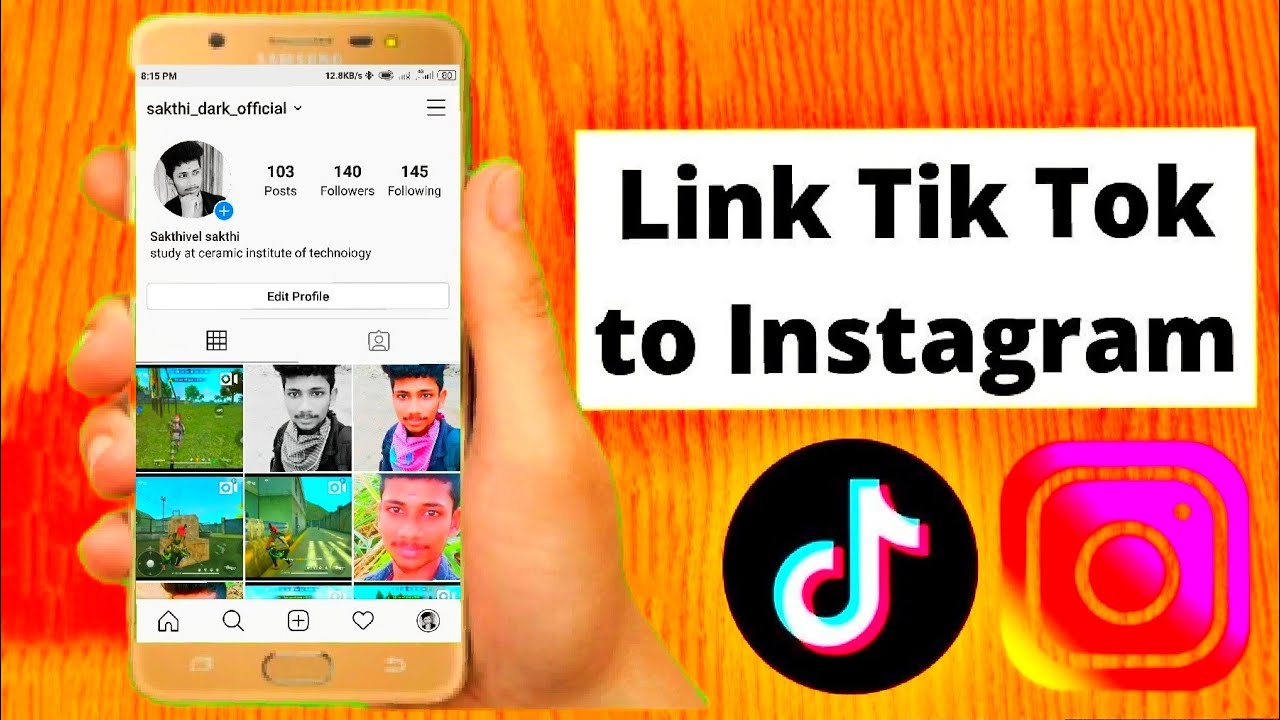The image appears to be a screenshot, possibly taken from a computer or captured from an online source. It features an orange-yellow background with a vertical wood grain pattern, alternating between hues of orange and yellow. Emerging from the bottom left corner of the image is a hand, palm facing forward, holding a cell phone. The cell phone's screen, clearly visible, displays an Instagram profile.

On the Instagram profile, a circular profile picture shows a man with dark hair, suggesting his username is "Sock the Dark Official." Below the profile picture are several posts, with a mix of video game screenshots and personal photos of the man, who appears to be of Indian descent.

To the right of the phone screen, there's a large white rectangle featuring a bold, black text message: "Link TikTok to Instagram." Below this message is the TikTok symbol, a large black circle with a white letter 'T' inside. The Instagram symbol, characterized by a gradient of purple and pink and resembling a camera, is also present.